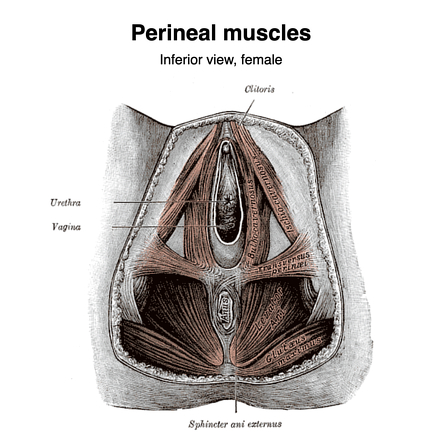This is a detailed anatomical drawing from a medical textbook, titled "Perineal Muscles, Inferior View, Female." The illustration presents a labeled, close-up view of the perineal region from beneath a female perspective, indicating the anatomical setup of the urethra, vagina, clitoris, and sphincter. The drawing primarily uses a grayscale palette with highlighted areas in a pinkish-orange hue to distinguish the muscles and tendons. The central area of focus is an oval shape, featuring a small black dot where the urethra is marked, a tiny white dot at the top labeled as the clitoris, and lines pointing to the respective locations of the vagina and sphincter. While the image does not delve deeply into intricate details, it serves as a general yet informative representation for educational purposes, helping viewers identify and understand these essential parts of the female pelvic anatomy.